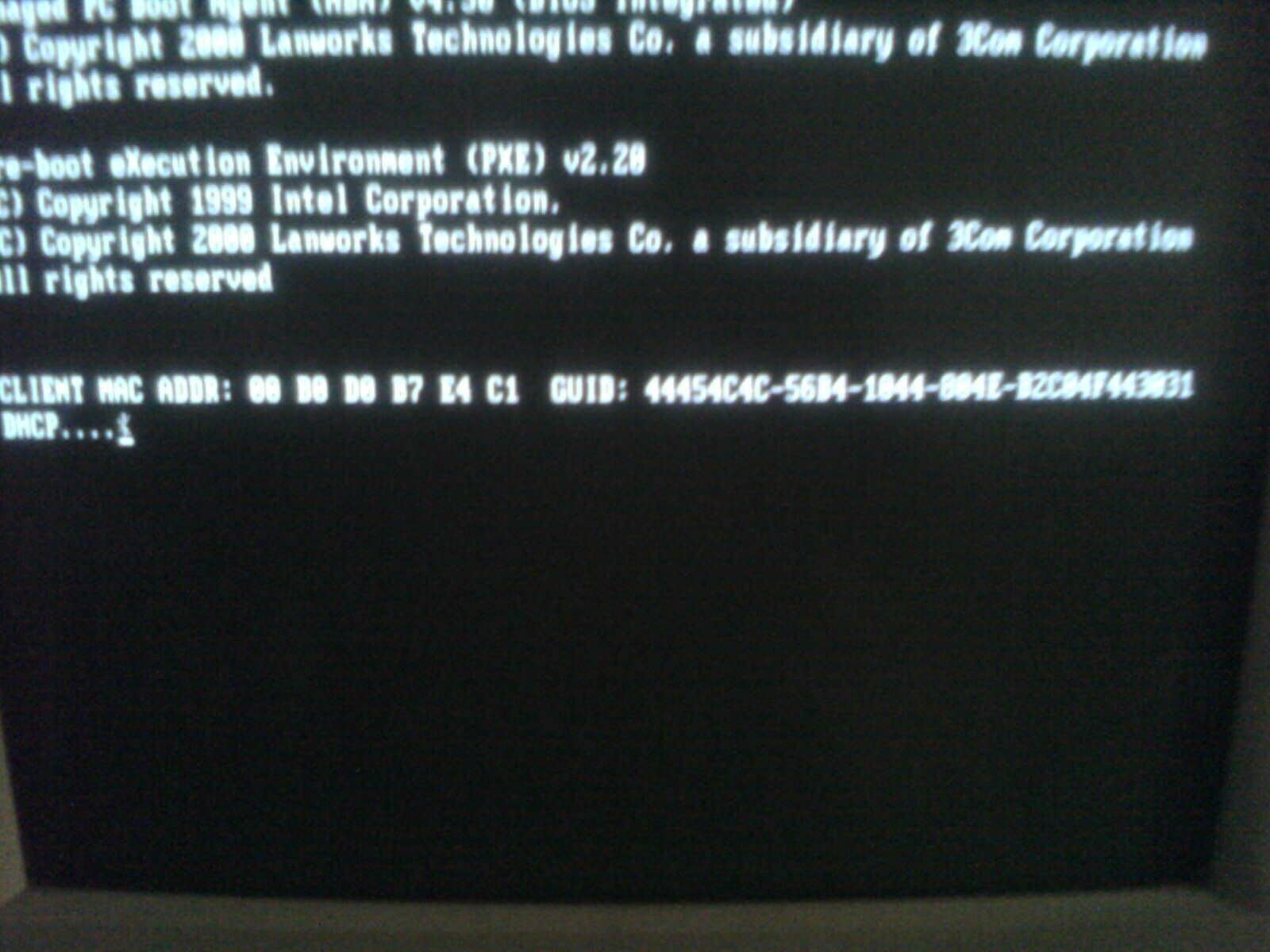This detailed image captures a close-up of an old computer monitor displaying a blurry and glary MS-DOS screen. The text is written in bright white letters on a black background, although the image quality makes the text difficult to read clearly. The top line reads, "Copyright 2000, Landworks Technologies Co., a subsidiary of 3Con Corporation, rights reserved." Below this, there's a space followed by "Boot Execution Environment (PXE) v2.20", and further down, "Copyright 1999, Intel Corporation. Copyright 2000, Landworks Technologies Co., a subsidiary of 3Con Corporation. All rights reserved." Additional lines include a client MAC address, but the details are hard to discern due to the image's blurriness. The monitor's gray frame is visible at the bottom, further emphasizing the dated appearance of the hardware.